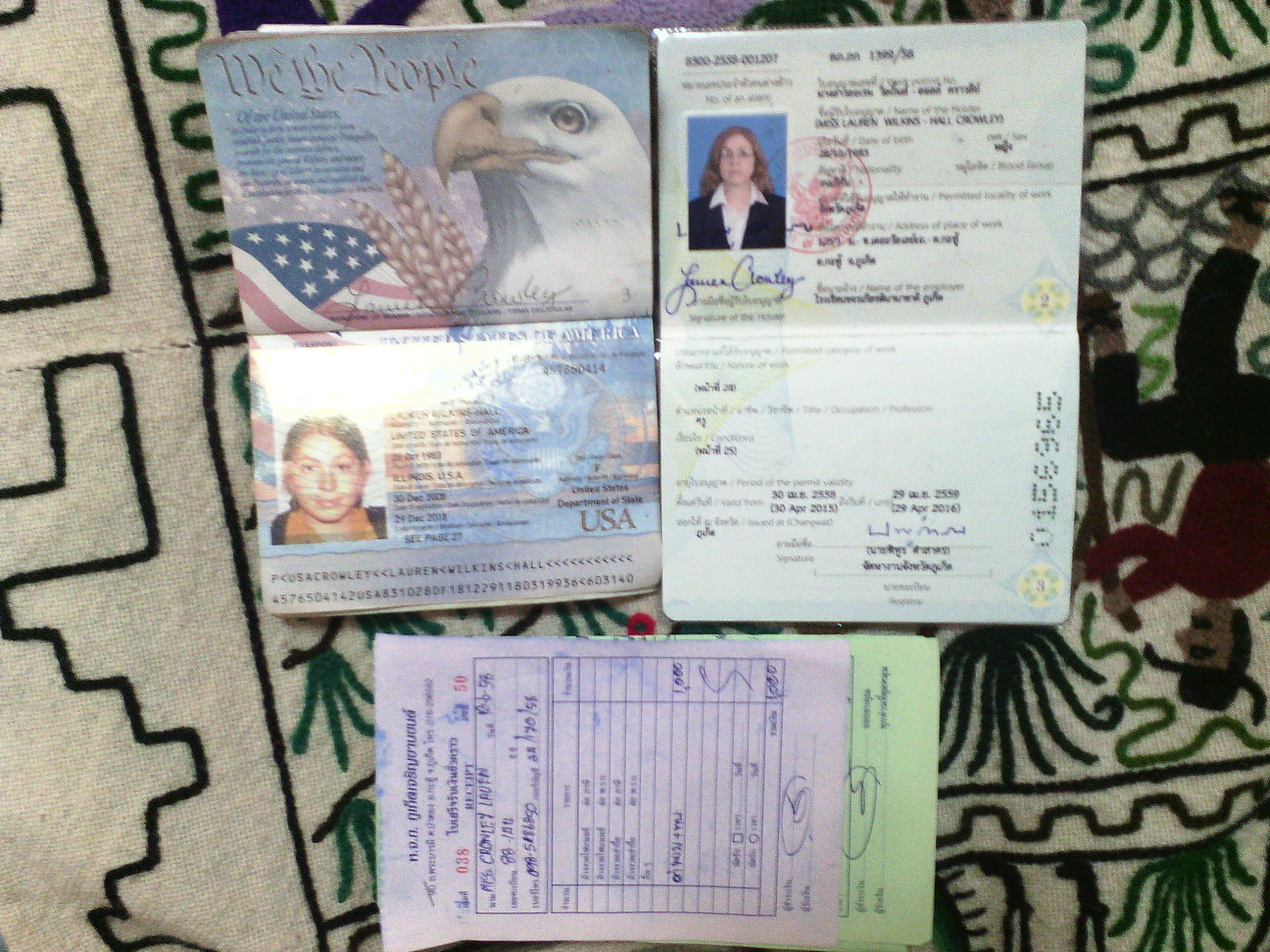The image showcases a young woman's passport and potentially other immigration papers, all laid out on a white carpet with black line designs. On the left is an open American passport displaying the text "We the People" alongside a bald eagle, an American flag, and grain imagery, with "USA" marked in the lower right corner. The woman's photo on this passport shows her with brown hair, wearing a black shirt and an orange scarf. Next to the American passport is another document, possibly an identification form from a different country, which features a red stamp, a signature starting with "L and C," and the number 0156965 alongside yellow symbols labeled 2 and 3. In the woman's passport photo on this document, she has reddish hair and is dressed in a black suit coat over a white collared shirt. Below these documents is a purple paper overlapping a green paper with lots of small, unreadable text and a grid of information. The scene is set on a carpet decorated with abstract and farm-themed designs, including an upside-down image of a man working with what appears to be a Y-shaped water dousing rod among plants.